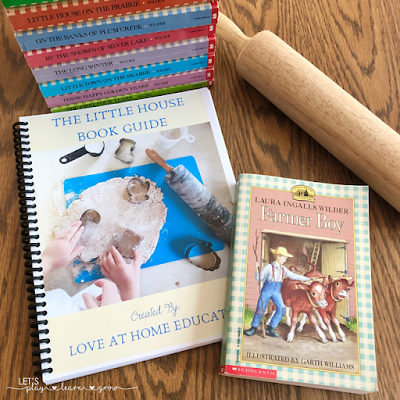The image features a collection of books and a rolling pin arranged on a light wooden table. To the upper left, there's a neatly stacked series of multi-colored books from the "Little House on the Prairie" series, showcasing various spine colors including orange, light blue, pink, and shades of blue. Towards the center left, prominently displayed, is a spiral-bound cookbook titled "The Little House Book Guide." The cover illustrates a scene of someone rolling out dough with a rolling pin and metal cutouts, alongside the partial text "Love at Home Education." Adjacent to this cookbook, to the right, lies the book "Laura Ingalls Wilder, Farmer Boy," depicting a boy in overalls and a straw hat standing next to two cows, set against a checkered background. Additionally, a lighter wood rolling pin is placed in the upper right corner of the image.